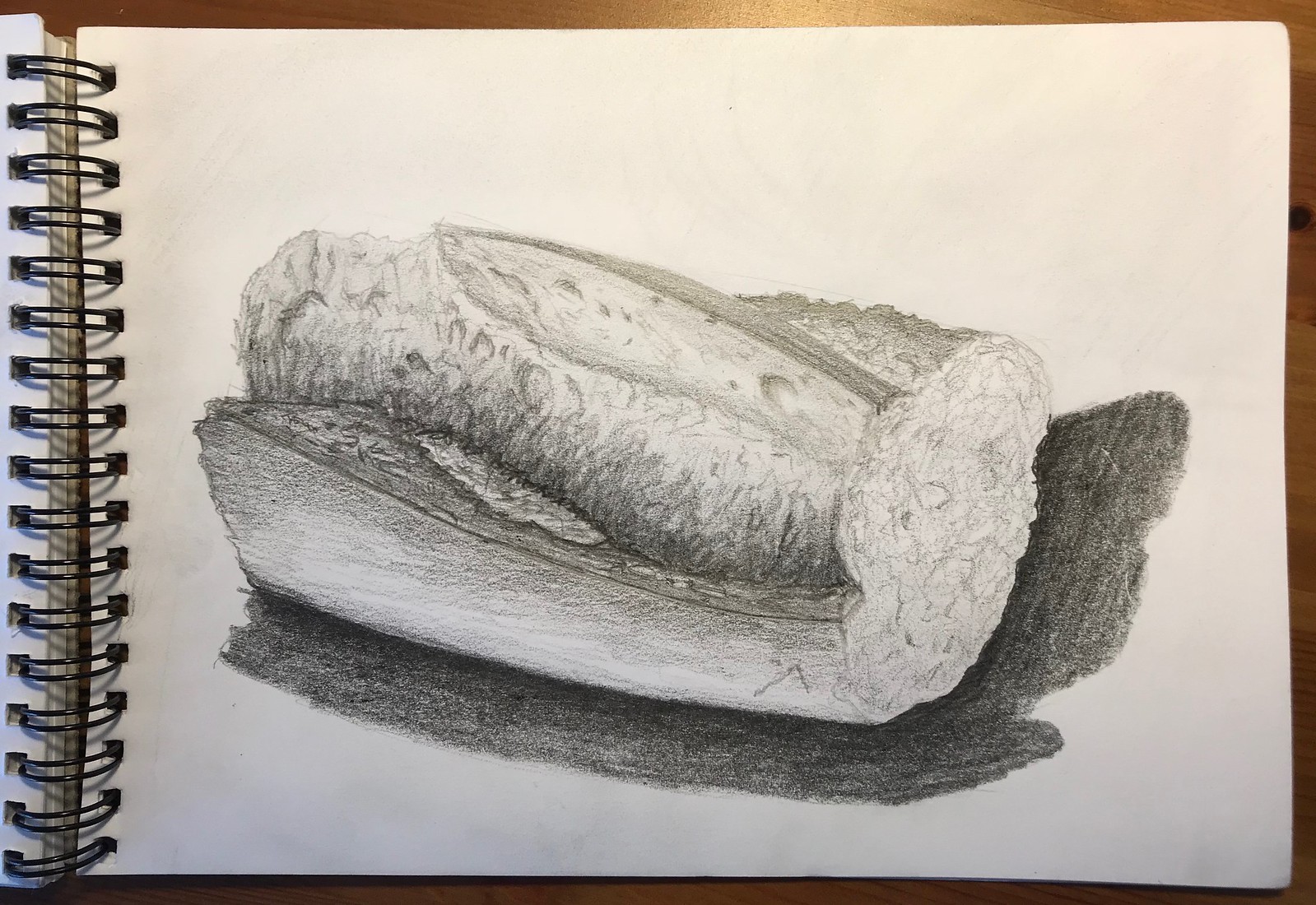In this highly detailed image, a spiral-bound sketchbook, open to a page, lies sideways on a wooden tabletop, with its black spirals visible along the right-hand side. The white sketch paper features a meticulously drawn pencil and colored pencil illustration of a loaf of bread that has been cut in half. The loaf, resembling French bread, is unevenly shaped and displays intricate ridges and imprints. A prominent diagonal line runs from the upper left to the lower right, emphasizing the texture and crust of the bread, which is portrayed with exceptional shading to capture its crusty appearance and holes from baking. A shadow extends from the bottom of the loaf to the right corner where it has been cut, rendered in dark gray to enhance the dimensionality. The tabletop's brown surface subtly frames the sketch, peeking out from the top right, down the left side, and beneath the book, grounding the entire scene.